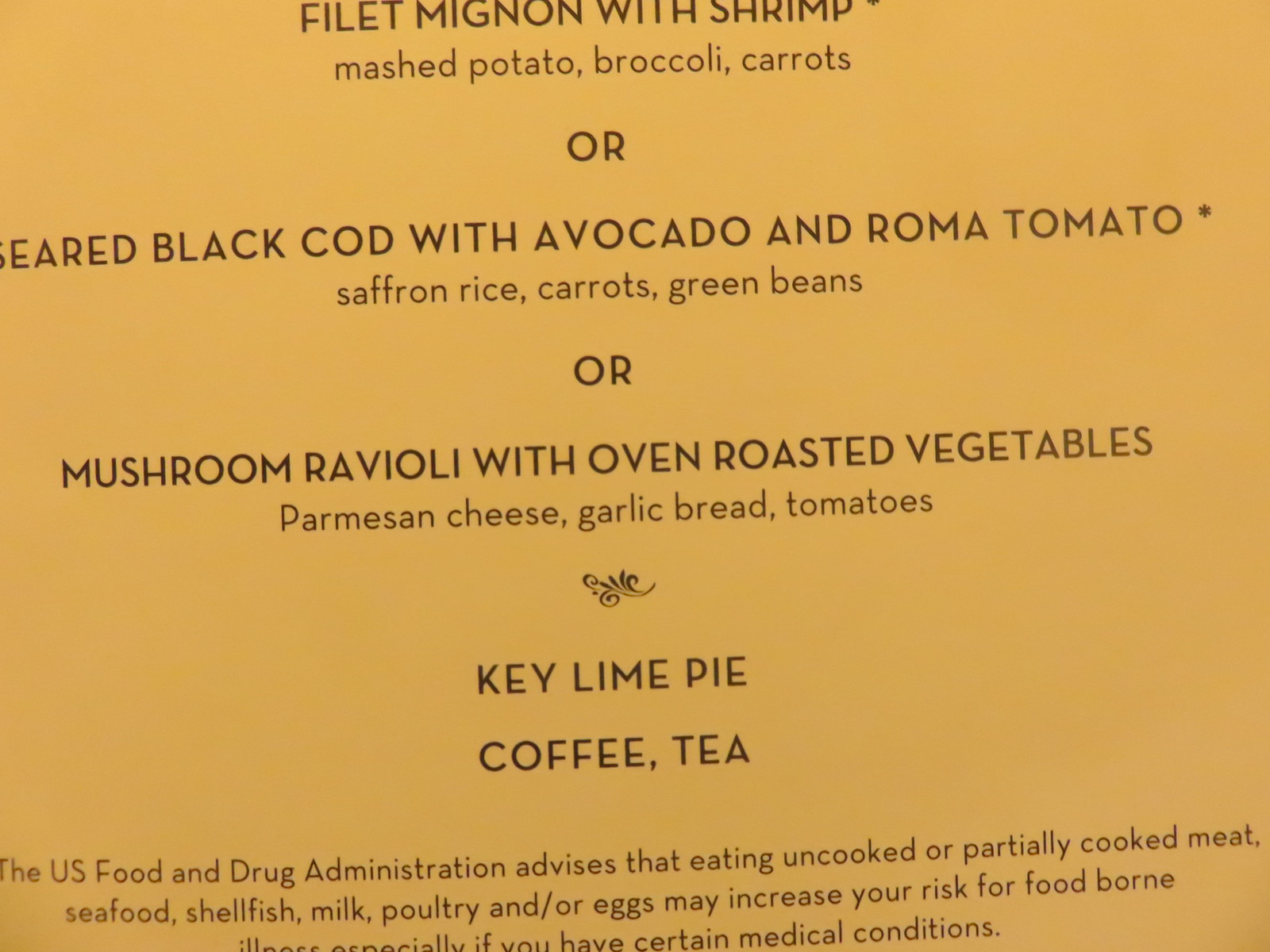This image depicts a section of a restaurant dinner menu on a yellowish background. At the top, the partially cut-off title reads "Filet Mignon with Shrimp," followed by its accompaniments: mashed potato, broccoli, and carrots. Alternatively, the menu offers "Seared Black Cod with Avocado and Roma Tomato," which includes saffron rice, carrots, and green beans, marked with an asterisk. Another option listed is "Mushroom Ravioli with Oven-Roasted Vegetables," featuring Parmesan cheese, garlic bread, and tomatoes. At the bottom of the menu, desserts and beverages are highlighted with "Key Lime Pie, Coffee, Tea" in all caps. A footnote with the asterisk mentions: "The U.S. Food and Drug Administration advises that eating uncooked or partially cooked meat, seafood, shellfish, milk, poultry, and or eggs may increase your risk for foodborne illness, especially if you have certain medical conditions." The text is black, making it readable against the yellow background.